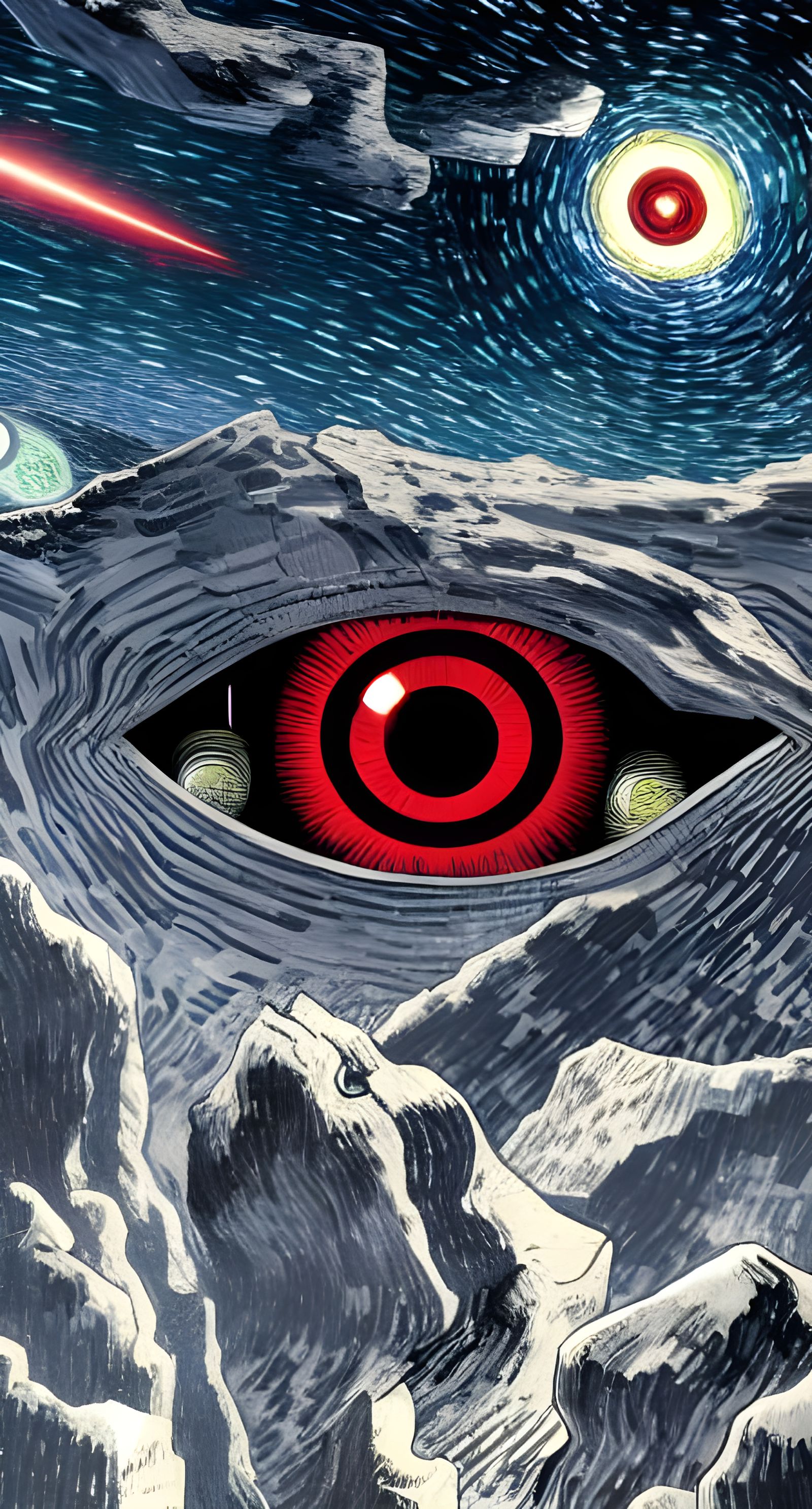The image vividly combines surreal and abstract elements, presenting a dreamlike cosmic scene. At the top, there is a time-lapse depiction of the night sky, featuring numerous stars with motion trails, a meteor streaking through, and a couple of asteroids, alongside a bright globe of light which could be interpreted as the moon or a distant planet, enveloped in a red halo resembling an ethereal eye. Below this celestial display, the composition transitions to a jagged, rocky landscape resembling a lunar surface. Central to the image is a prominent, glaring eye embedded in a rocky crevice. This eye, with its red ringed iris and black pupil, is accented by two green dots and appears to peer out ominously from the rock. The lower section of the image further details more craggy cliffs and an alien figure camouflaged among the rocks, possessing noticeable eye and mouth features. This composition masterfully blends realistic astronomical elements with surrealist and impressionist artistry, creating a captivating and otherworldly visual experience.